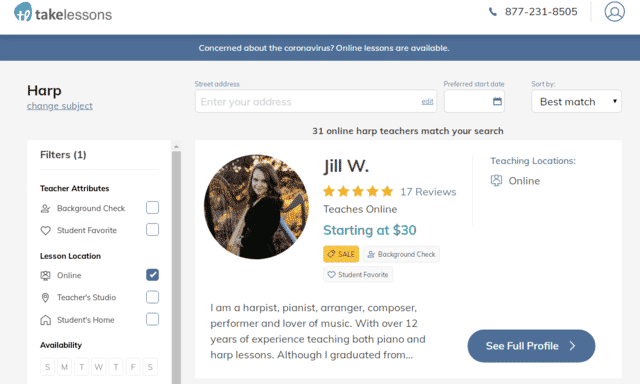This image is a detailed screenshot from the TakeLessons website. At the top, there's a prominently displayed phone number (877-231-8505) for inquiries. A tab reveals a circular placeholder for users to upload their profile images upon creating an account. Below, a blue banner highlights the site's response to COVID-19 with the message: "Concerned about the coronavirus? Online lessons are available." 

Continuing down the left-hand side, various filters are displayed, starting with "HAARP" under which it says "change subject." The first filter category, "Teacher's Attributes," mentions factors like background checks and student favorability. Next, "Lesson Locations" provides options such as "Online," "Teacher Studio," or "Student's House," with the online option pre-selected. The "Availability" filter lists the days of the week abbreviated as SMTWTFNS—Sunday through Saturday.

In the middle of the screen, within the main content area, a profile for Jill W. is shown. It states that 31 HAARP teachers are available online. Jill W.'s profile specifies that she offers online lessons starting at $30 per hour, is currently running a sale, has completed a background check, and provides lessons exclusively online.